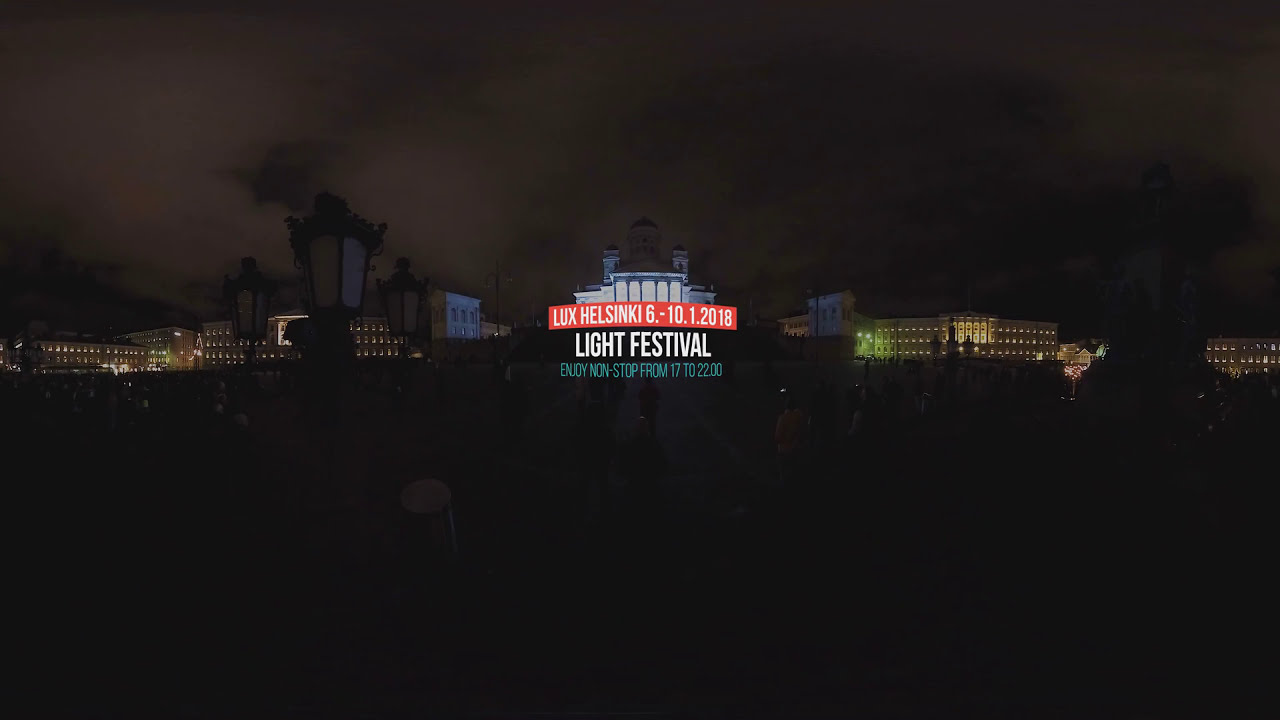The photograph, taken at night, depicts a panoramic view of a darkened outdoor venue, with a cloudy sky adding to the overall dimness. In the distance, several lit windows from two to three-story buildings, possibly hotels, are visible. Despite the street lights being unlit, the scene is partially illuminated by the green lights outside one of the buildings. Palm trees are situated in the left midsection of the frame. The center of the image features an illuminated advertisement that reads, "Lux Helsinki, 6-10, 1, 2018 Light Festival. Enjoy non-stop from 17 to 2200." Additionally, there are numerous people discernibly walking around at this outdoor Light Festival, contributing to a lively yet subdued atmosphere.